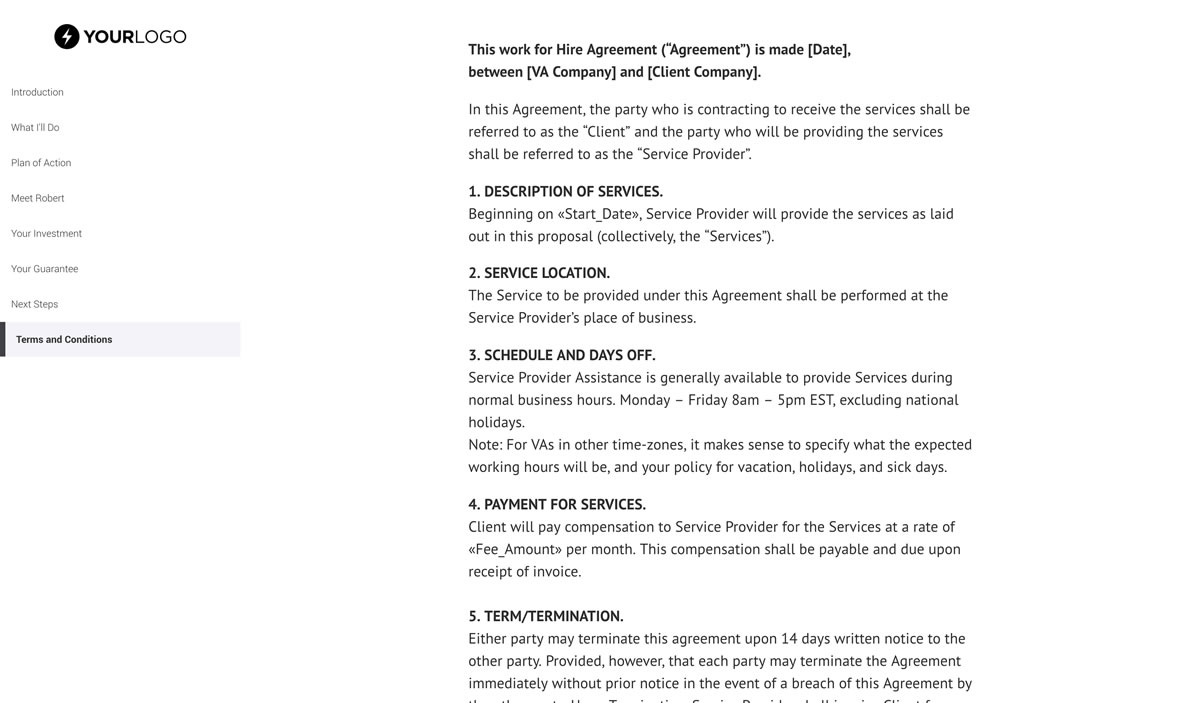This image is a detailed screen capture of a business agreement documentation, specifically a work-for-hire contract. The left side of the image features a logo represented by a black circle containing a white lightning bolt, accompanied by the text "Your Logo." The word "Your" is rendered in bold black font, while "logo" is in a standard black font.

The document is organized into various sections, each headed in bold black text: 

- **Introduction**
- **What I’ll Do**
- **Plan of Action**
- **Meet (likely a placeholder indicating a name, "Robert")**
- **Your Investment**
- **Your Guarantee**
- **Next Steps**

Bordering and highlighting these sections is a gray box with a black line adjacent to it. Below this is a header indicating the **Terms and Conditions** of the agreement.

At the top, the document is titled **Work for Hire Agreement**. It starts with, "This work for hire agreement is made," followed by placeholders for the date, the company, and the client company in brackets. Within the agreement, the client is identified as the party receiving the services, while the service provider refers to the party delivering the services.

The agreement includes several detailed clauses:

1. **Description of Services**: Beginning on the start date, the service provider will offer the outlined services, collectively referred to as "the services."
2. **Service Location**: These services will be performed at the service provider's place of business.
3. **Schedule Days Off**: The service provider's assistance is generally available during normal business hours, Monday through Friday, 8 a.m. to 5 p.m. Eastern Time, excluding national holidays. There’s a note indicating the importance of specifying expected working hours and policies for vacations, holidays, and sick days, especially for VAs in different time zones.
4. **Payment for Services**: Clients agree to compensate the service provider at a specified monthly rate, payable upon receipt of invoice.
5. **Terms/Termination**: Either party may terminate the agreement with 14 days written notice. Immediate termination without prior notice may occur in cases of agreement breach.

The document cuts off before completing the section on termination, indicating further details exist beyond the captured image.